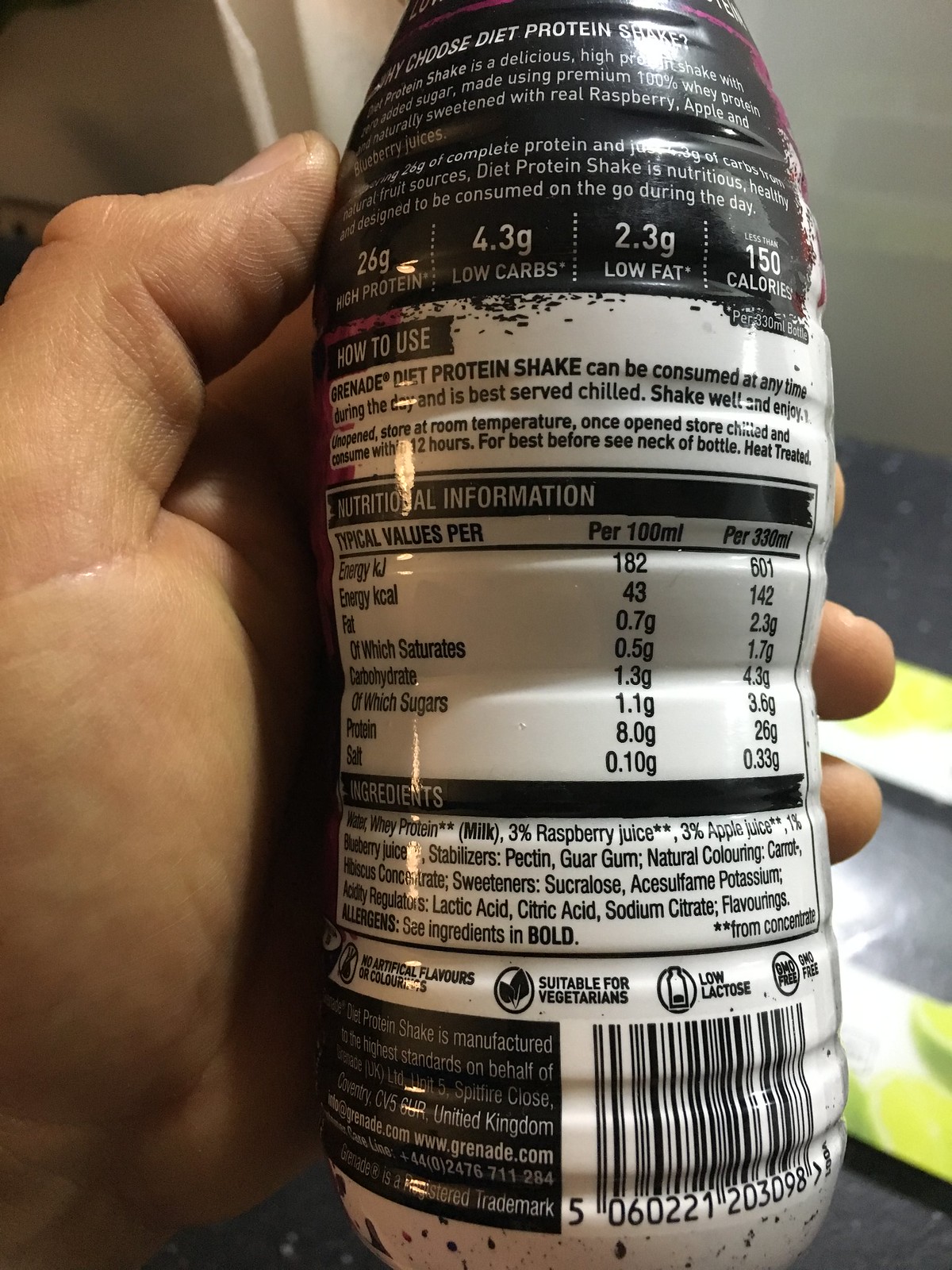In this photograph, a Caucasian person's hand is prominently featured holding a protein shake bottle. The hand is positioned such that the palm and thumb are visible on the left side of the bottle, while three fingertips securely grasp the right side. The focus is on the back label of the bottle, which clearly displays a variety of product information in white font.

At the top of the label, the text reads, "Choose diet protein shake." Below this headline, the nutritional benefits are listed in detail: "26 grams of protein, 4.3 grams low carbs, 2.3 grams low fat, 150 calories." Further instructions on how to use the product are also included: "Grenade diet protein shake can be consumed at any time during the day and is best chilled. Shake well and enjoy. Once opened, store at room temperature. Unopened, store at room temperature. Once opened, store chilled and consume within 12 hours. For best before, see neck of bottle, heat treated." 

Additionally, the nutritional information and ingredients are mentioned on the label, though they are not fully legible in this shot. The scene is set against a black table adorned with some indistinct yellow and white line items resting behind the bottle, adding contrast to the image. Overall, the photograph sharpens the viewer's focus on the hand holding the detailed dietary supplement while providing a glimpse into the background context.